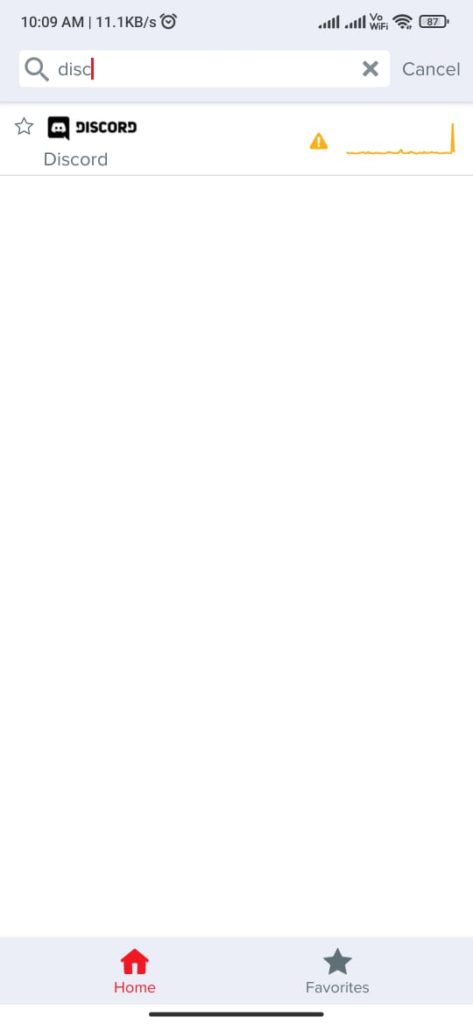The image depicts a screenshot likely taken from a cell phone. In the upper left corner, displayed against a light gray banner, the time is shown as 10:09 a.m. in black text. To the right of the time, the data usage indicator reads 11.1 KB/s. An icon of an alarm clock is also visible, followed by fully lit bars indicating strong network reception. The Wi-Fi icon is active, and the battery level is at 87%.

Below these indicators, there is a white search bar with a magnifying glass icon on the left side. The letters "DISC" appear in the search bar, accompanied by a red mouse icon. On the right side of the search bar, the word "Cancel" is visible.

Further down, the icon for the Discord app appears, alongside the word "Discord" in bold black text. At the bottom of the page, another light gray banner houses several icons. There is a red house icon with the word "Home" in red text below it. To its right is a black star icon with the word "Favorites" in gray text underneath.